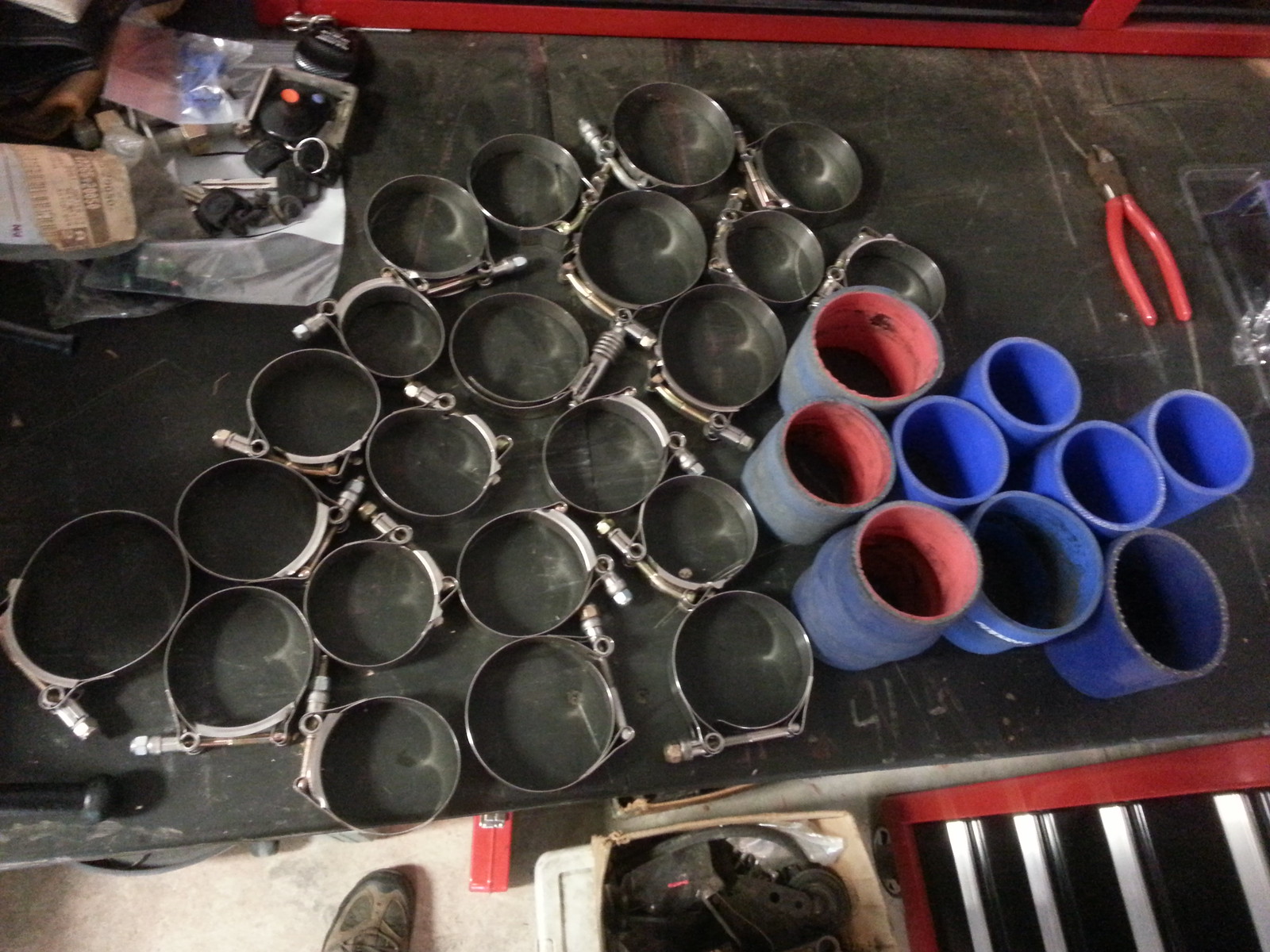The image is a color photograph taken from a first-person perspective, looking down at around a 45-degree angle onto a black workbench. The workbench, which appears to have a rubberized texture with visible wear and damage, is scattered with an assortment of tools and materials. In the bottom left of the image, the left foot of the person taking the photo is visible, clad in a brown shoe with some black accents.

On the left side of the workbench, extending to the right, there is a collection of stainless steel pipe clips. Each clip has a nut and bolt or screw on one part of the circumference, designed to tighten around a pipe fitting. Toward the top left, there are some indistinct items piled on top of each other, possibly tools or fixings used for DIY projects.

To the right of the pipe clips, there are several offcuts of pipes in various shades of blue. Six pipes on the right are blue both inside and out, while three pipes on the left are blue on the outside and red on the inside. Additionally, a pair of needle-nose pliers with red rubberized handles, pointing downwards to the edge of the workbench, is situated on the right side.

In the top right corner of the workbench, there is also a set of keys with silver rings, laying on top of a piece of white paper. Towards the bottom right, a red toolbox with black cabinets and silver handles is partially visible, along with a red object beneath the workbench. Scattered around the workbench are remnants like sawdust and other small debris, indicating recent use and material cutting activities.